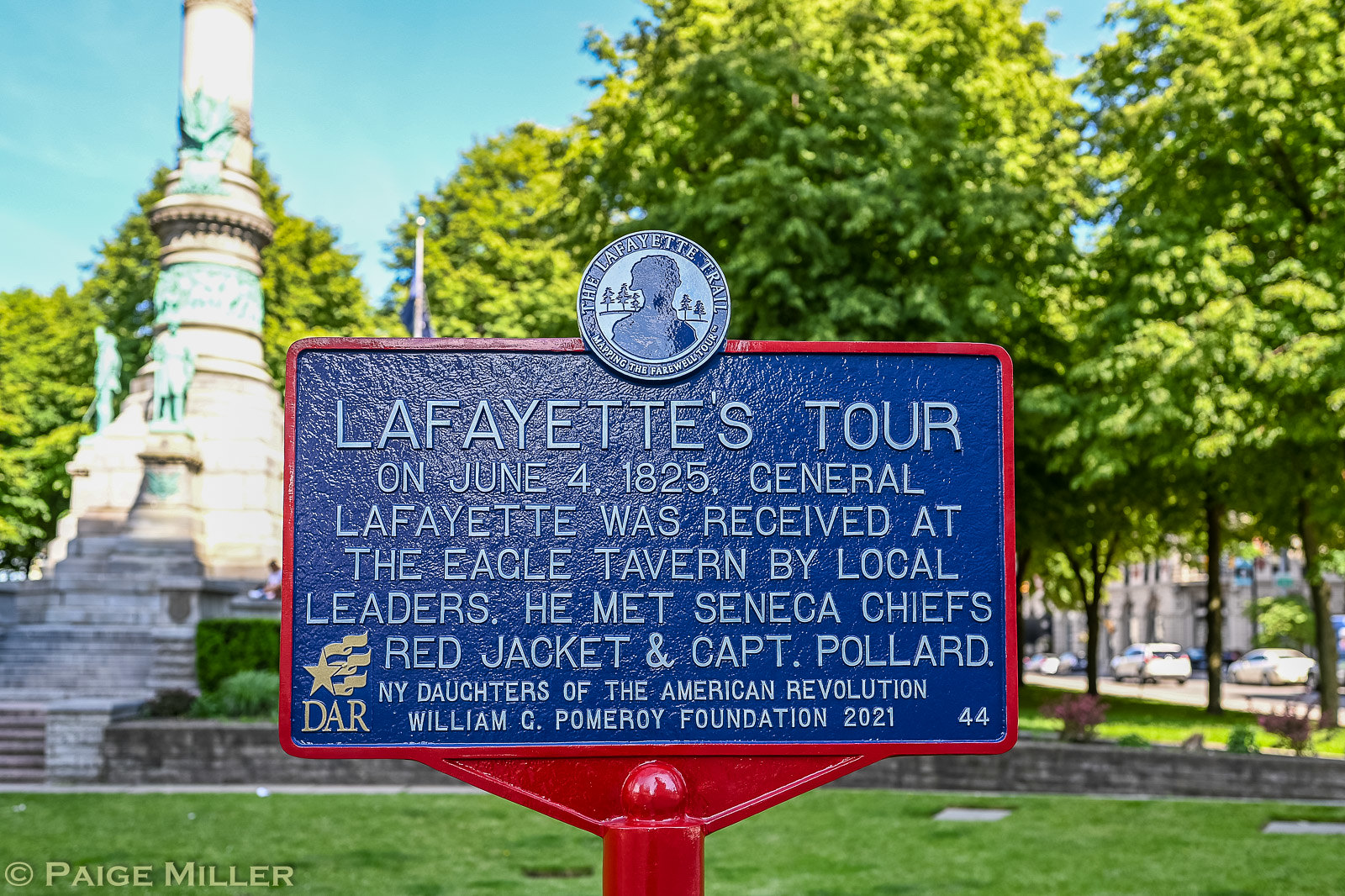This is a color photograph of a historical marker set in a park. The marker features a red border and a blue central panel with white raised text. At the top of the marker, it displays the seal of "The Lafayette Trail" followed by the title, "Lafayette's Tour." The inscription details that on June 4th, 1825, General Lafayette was received at the Eagle Tavern by local leaders, where he also met Seneca Chiefs, Red Jacket, and Captain Pollard. Below the main text, in smaller print, it notes the sponsors: NY Daughters of the American Revolution and the William G. Pomeroy Foundation, 2021. The Daughters of the American Revolution (D.A.R.) logo appears in the bottom left corner. The sign is mounted on a red post. In the background, there is a green lawn with an obelisk-like stone monument positioned towards the right. Trees are visible from the center to the right, and there is also a street with cars on the lower right.